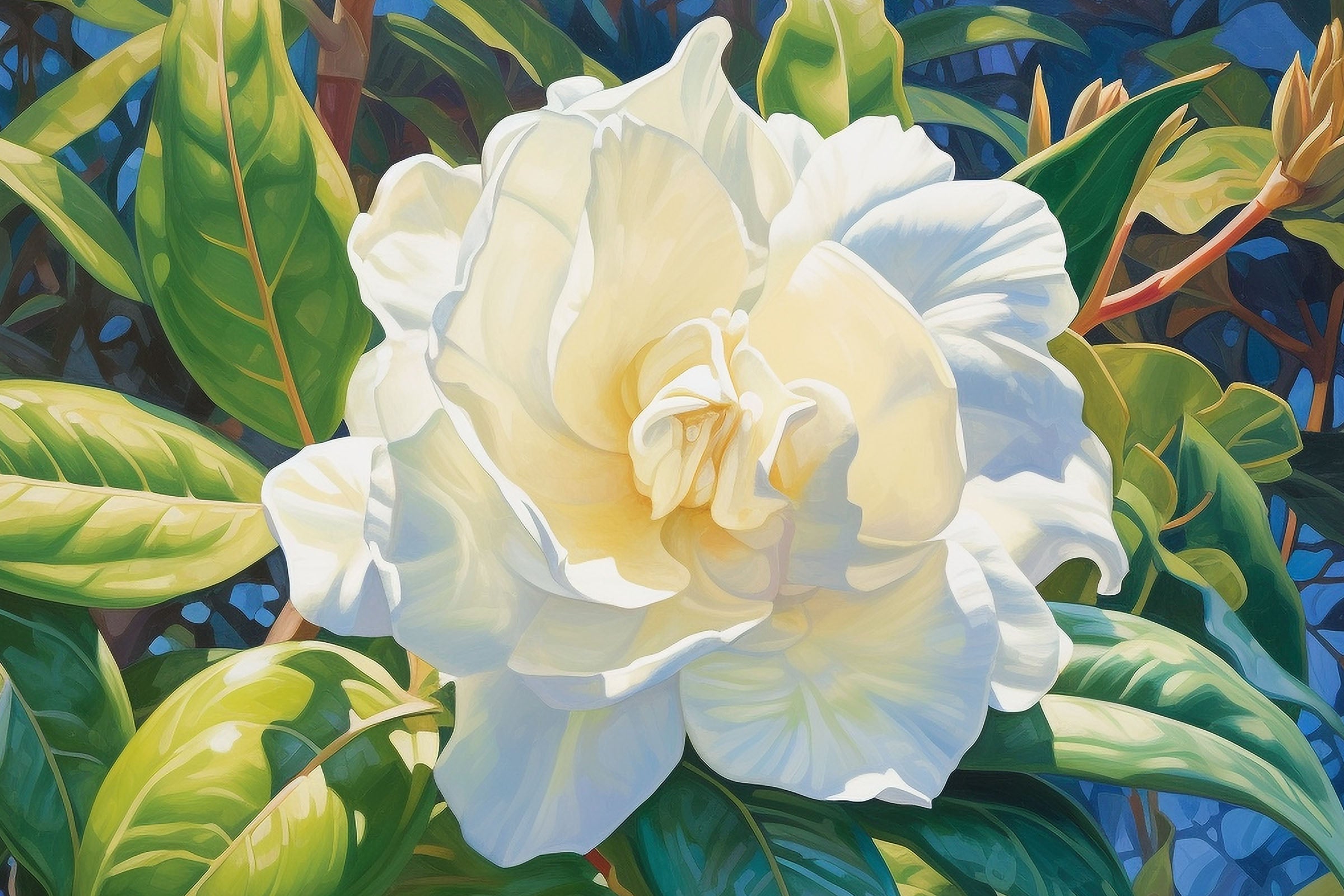This artwork, likely a modern painting from the 2000s, features a striking white flower that resembles a camellia or rose, fully blossomed and positioned at the center of the image. The petals exhibit subtle shifts in color, moving towards a cream hue at the center and displaying a faint bluish tint on the outer edges due to the sunlight. Surrounding the central flower are numerous green, teardrop-shaped leaves with brown center veins, introducing fine details to the composition. On the upper right corner, several flower buds are visible, suggesting new blooms are on the way. The background is enriched with purple leaf-shaped patterns, while yellow highlights on some leaves evoke a sense of daylight, contributing to the painting's realistic yet artistic and modern feel.